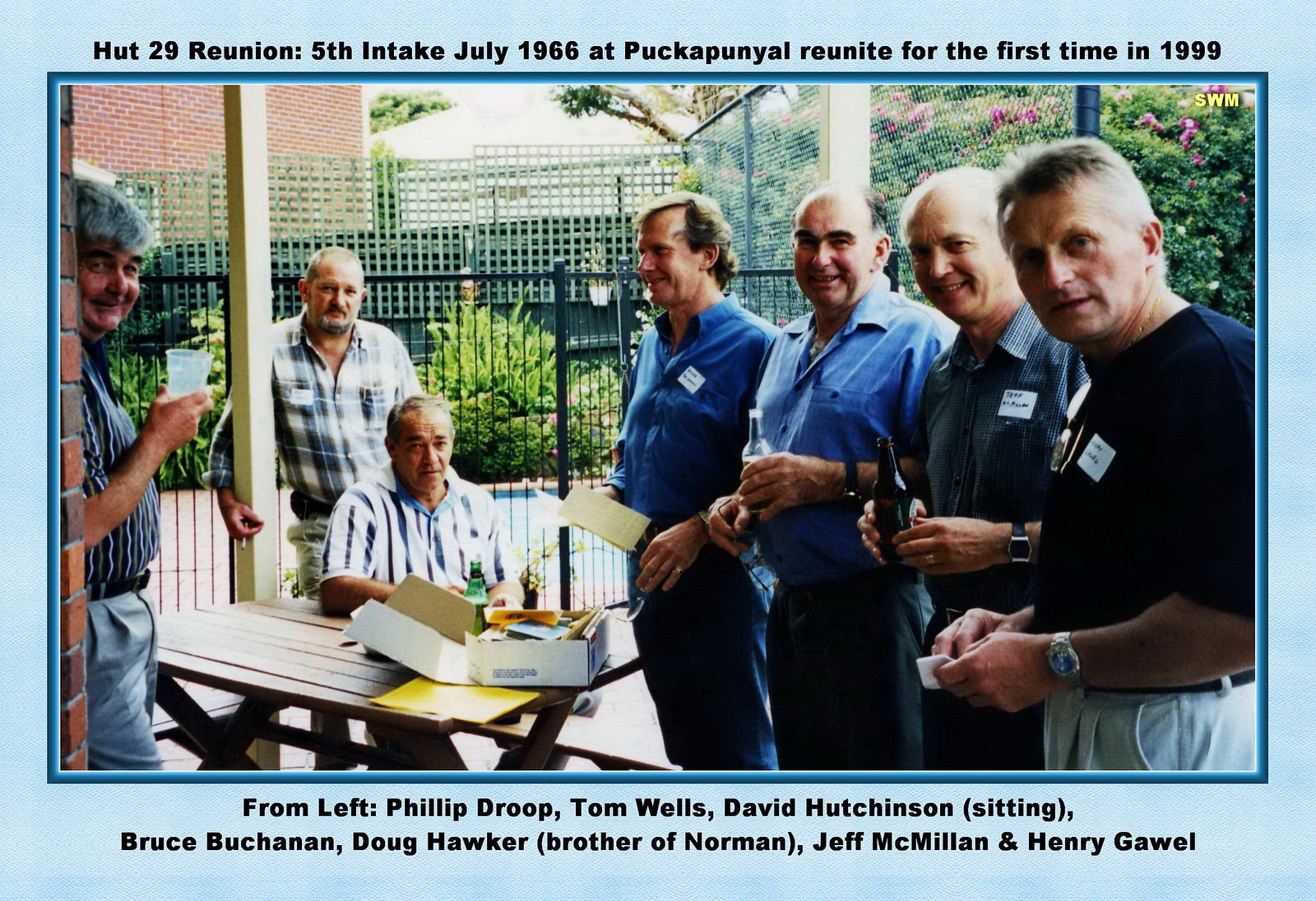This is a detailed photograph taken outdoors featuring a group of elderly gentlemen presumably at a military reunion. The men are gathered in a lush garden area with green trees, bushes, and pink flowers visible in the background, and a red brick building and a fence also part of the scenery. One man is sitting near a table while the others are standing or leaning, many holding bottles of beer. The setting appears to be a patio, possibly within a park. At the top of the image, a blue border frames the text: "Hut 29 Reunion, 5th Intake, July 1966 at Pucapinel Reunite for the first time in 1999." The bottom of the photo lists the names of the men from left to right: Philip Droop, Tom Wells, David Hutchinson (sitting), Bruce Buchanan, Doe Hawker (brother of Norman), Jeff McMillan, and Henry Galwell. The gathering captures a moment of camaraderie and nostalgia among the older men, one of whom appears to be of Asian descent while the rest seem white.